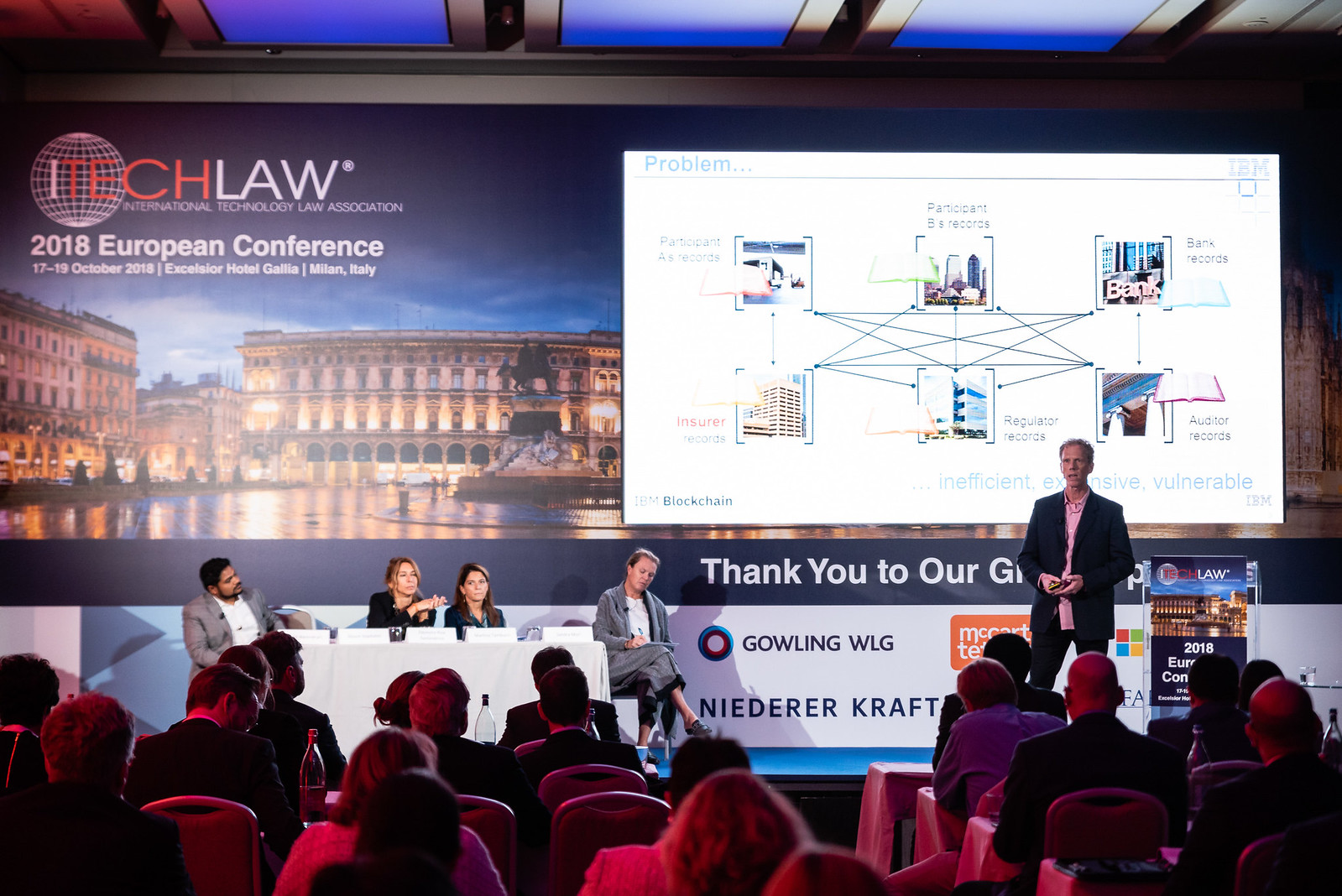The full-color, horizontally rectangular photograph captures an indoor scene at the 2018 iTech Law European Conference held from October 17-19, 2018, in Milan, Italy. The image depicts a large conference room illuminated by blue ceiling lights with tiles. At the forefront, several attendees of diverse ages and backgrounds are seated with water bottles placed in front of them on tables or trays. Up on the stage, five individuals are visible; four are seated behind a white table, while one stands giving a presentation. A large projected screen with a white background displays the conference logo, which includes a globe and the text "iTech Law," along with the event details. The presenter appears to be discussing business growth, possibly in German, and is seen thanking the audience. The room's darker atmosphere is interrupted by colorful lights that cast a reddish hue on the participants. To the upper left of the image, the screen features an image resembling Italy's iconic Coliseum, enhancing the context of the conference's location in Milan.